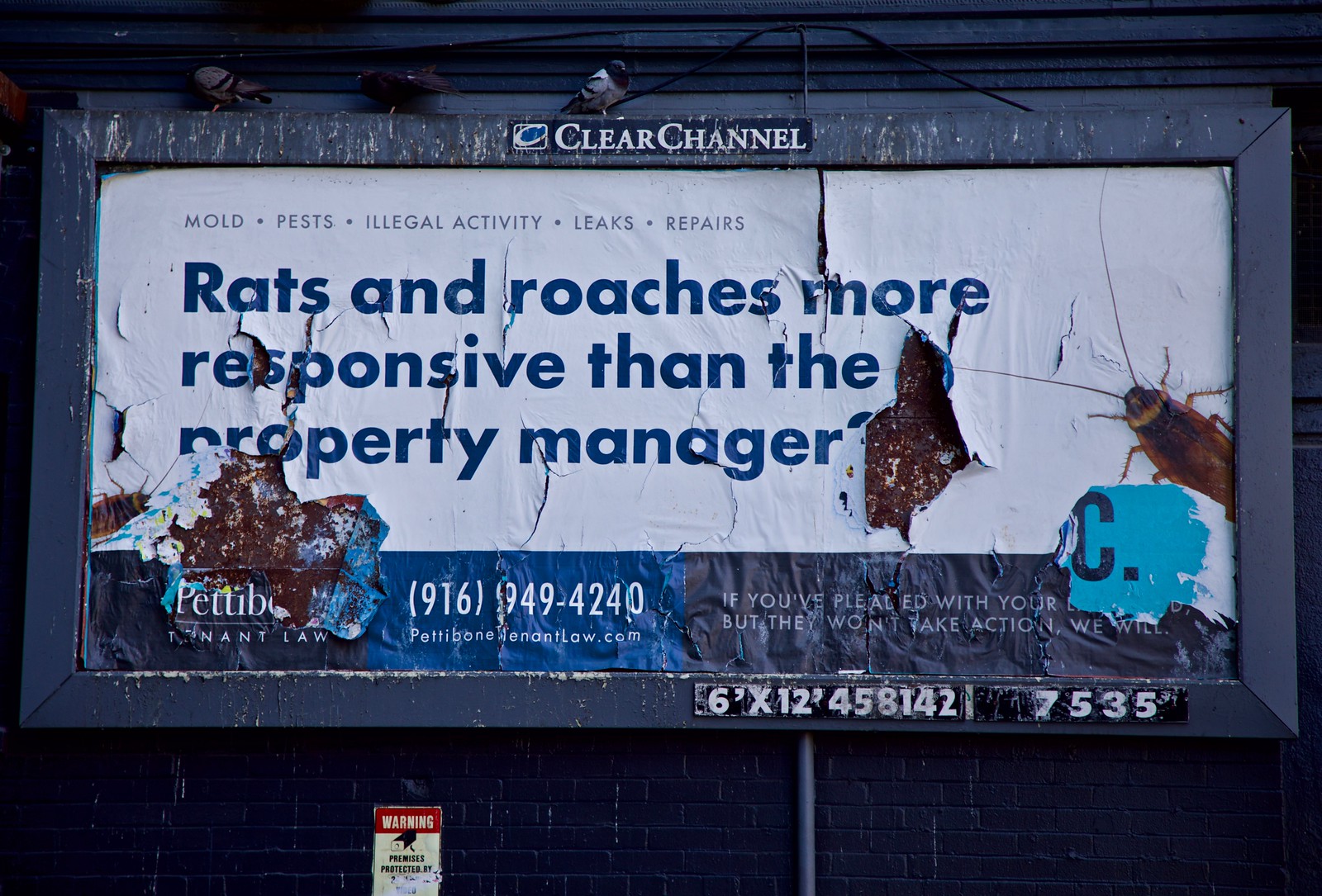The image features a rectangular billboard mounted on the side of a dark blue painted brick building. The top of the billboard reads "Clear Channel," indicating the maintenance company. The upper two-thirds of the billboard, with a distressed white background riddled with holes and tears that reveal patches of brown beneath, has blue lettering stating, “Molds, pests, illegal activity, leaks, repairs, rats and roaches more responsive than the property manager.” The fragmented state of the billboard adds a layer of irony to its message advocating for tenant rights. In the bottom right corner of this section, there's a visible top half of a cockroach. The lower third of the billboard is blue, featuring a phone number, "916-949-4040," in white. Perched atop the billboard are several pigeons, and a slate gray pipe is seen emerging from the bottom, slightly off-center to the right. The entire scene conveys a sense of neglect and decay, emphasizing the billboard's critique of property management.